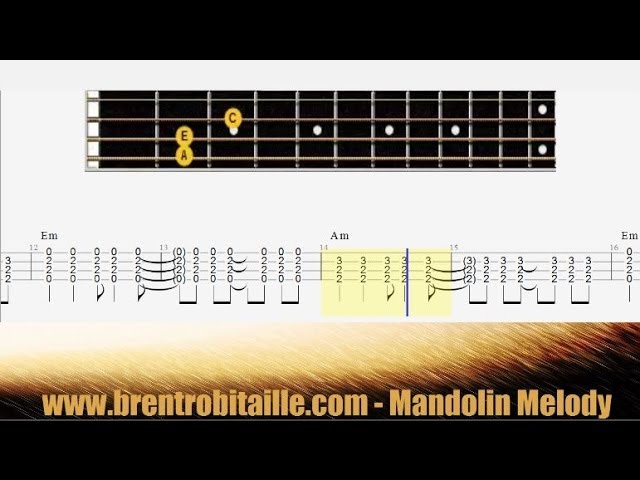The image is an instructional poster or screenshot from a tutorial guide, aimed at teaching how to play a melody on the mandolin, a small stringed instrument. The poster features a black background at the top with the website www.brentrobitaille.com prominently displayed. Below the website are graphics depicting a portion of the mandolin's fretboard, highlighting the finger positions for playing specific notes labeled A, E, and C. Further down, the poster transitions to a white background displaying musical notes that indicate chord progressions or sequences to be played. The detailed visuals suggest that this snippet is part of a larger structured song, providing clear instructions on finger placement and musical notation to facilitate learning. The bottom of the image includes blurred graphics of sparks, adding a dynamic touch to the instructional content.